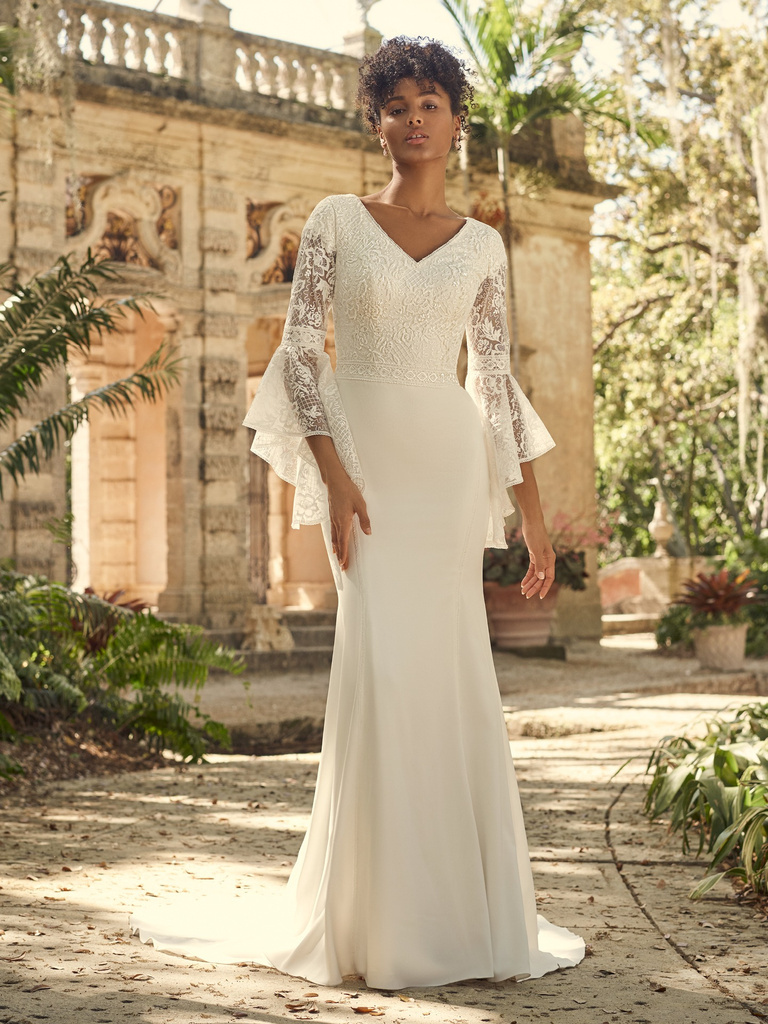In this professional portrait-oriented photograph, a young woman with a rich caramel mocha skin tone and tight curly hair pinned up is modeling a wedding dress. She stands on a sunlit cement pathway framed by greenery and palm trees, looking directly at the camera with a neutral expression. 

The wedding dress she models is long and sleek with a V-neckline and is adorned with lace from the waist up. The full sleeves of the dress transition into Victorian-style lace from the elbows down. The smooth, straight bottom of the dress extends into a train trailing behind her. The background features an old, elaborate white stone building partially visible amidst the foliage, suggesting a bright, sunny day emphasized by the shadows cast on the pathway.